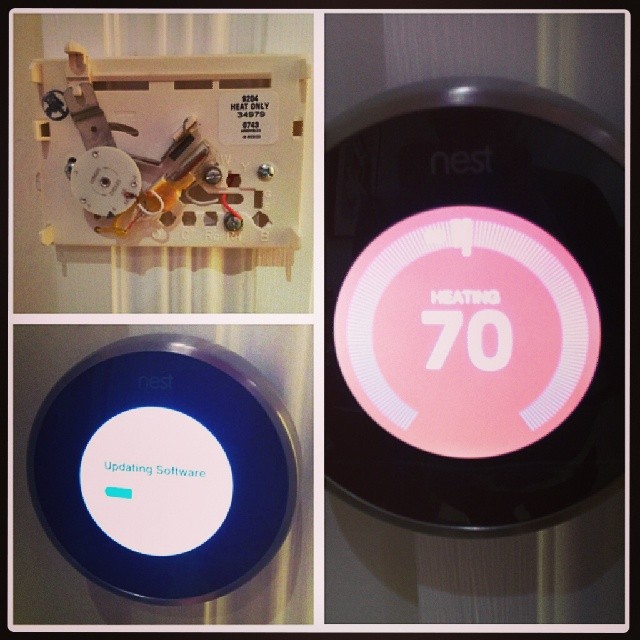The image is composed of three smaller images arranged in a square formation, depicting a digital smart thermostat mounted on a vertical striped wallpapered wall. The wallpaper is gray with white stripes running vertically.

- The top-left image shows the thermostat with its cover removed, exposing the internal components, including a mercury switch and a dial. The device is marked with the model number "9204, heat only, 34979."

- The bottom-left image features the disc-shaped thermostat intact. The display shows a white circular center with blue text that reads "updating software."

- The right-side image is a close-up of the thermostat's center display. The center circle is pink, with a white graduated arc around it. A white mark indicates the current setting. The text in the center reads "heating 70," indicating that the thermostat is actively heating to 70 degrees.

The detailed images collectively showcase different operational and physical aspects of the digital smart thermostat across various states.